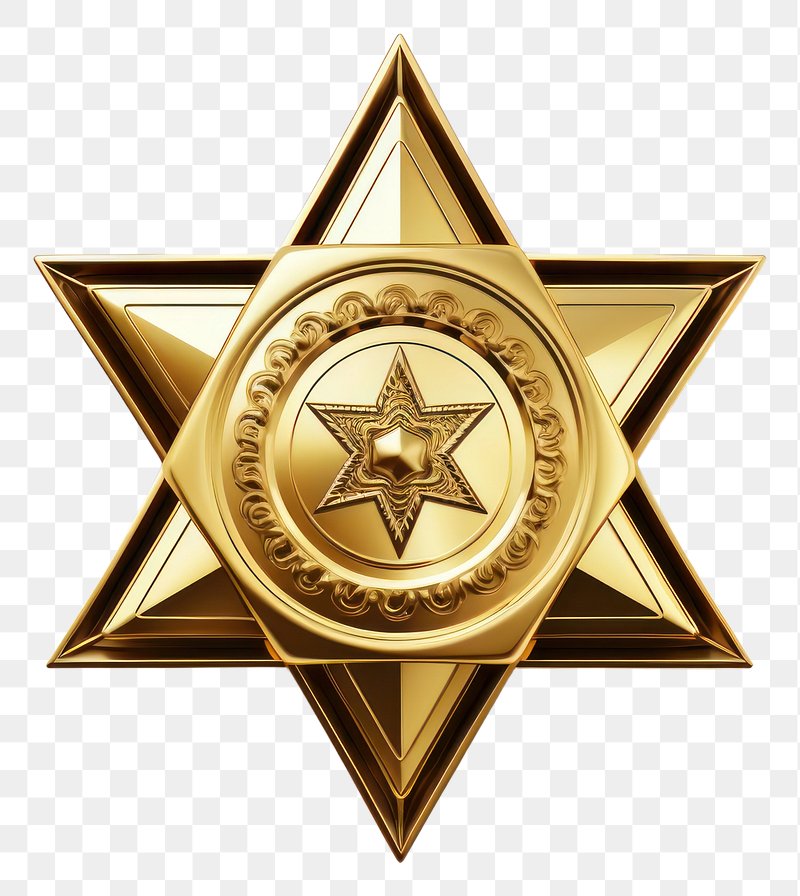This image features a gold star prominently displayed against a background that appears to be disintegrating from a pattern of blue and white squares. The star itself is quite intricate, boasting six sharply pointed sides. The outer edge of the star is gilded in gold, bordered by a thin layer of what looks like either black or brown. This border is further accentuated by two additional lines that add complexity to the design.

At the center of the star lies a hexagonal shape, adorned with an intricate floral pattern along its edges. Nestled within this central hexagon is another star, which also adopts a hexagonal form in its design, providing a visually captivating layer to the overall composition.